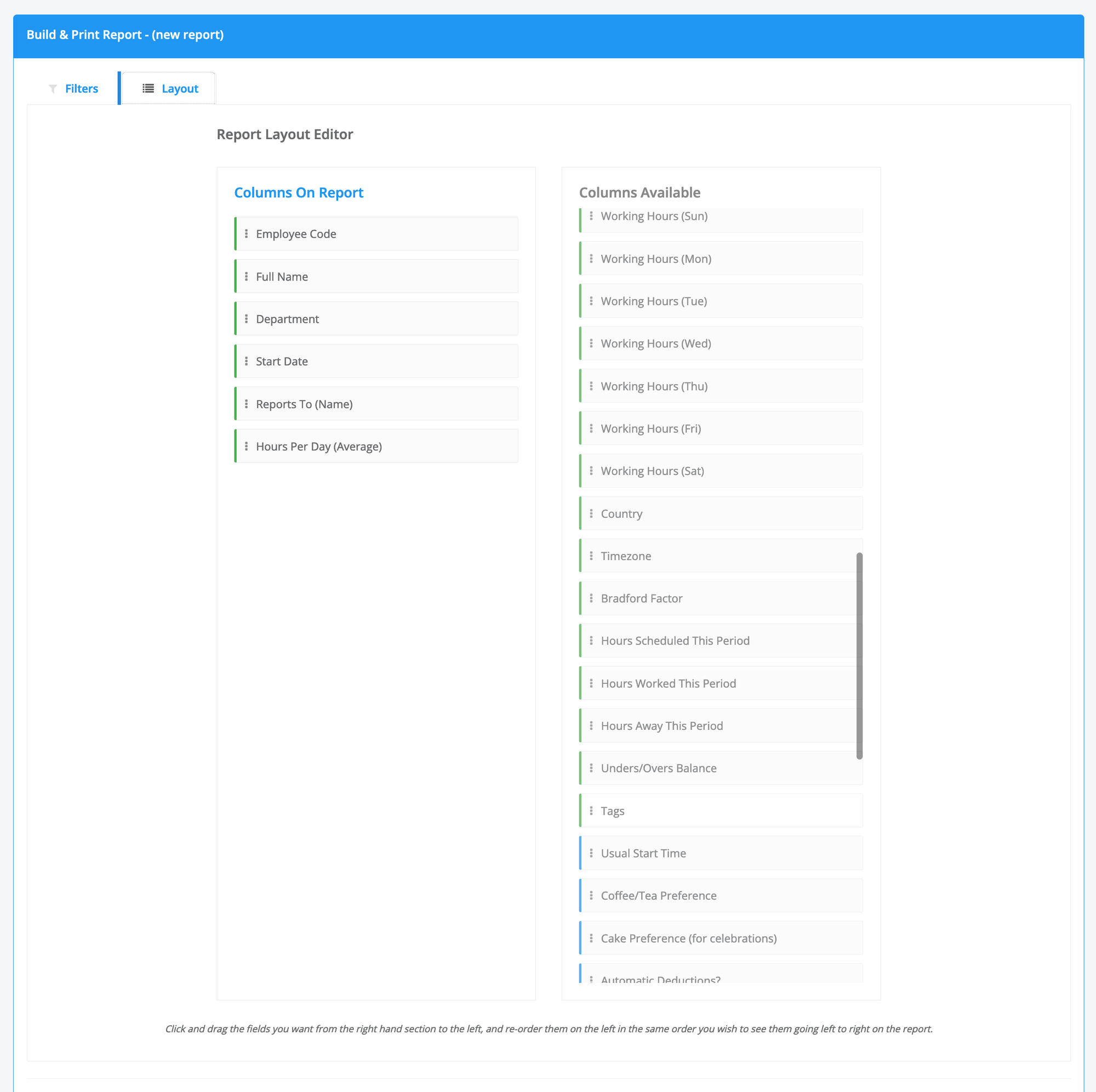The image depicts a computer screen featuring a detailed interface for building an InPrint report, with a blue border running across the top. In the upper left-hand corner of the border, white text reads "Build InPrint Report, New Report." Below this, two blue text tabs are visible: "Filters" and "Layout."

Just beneath these tabs, there is a vertical column on the left with a heading in black text labeled "Report Layout Editor." Under this, in blue text, the heading reads "Columns on Report," which lists six categories: Employee Code, Full Name, Department, Start Date, Reports to Name, and Hours Per Day Average.

On the right, another column is visible with the heading "Columns Available" highlighted in blue text. This column includes a comprehensive list of categories such as Working Hours Sunday through Saturday, Country, Time Zone, Bradford Factor, Hours Scheduled This Period, Hours Worked This Period, Hours Away This Period, Unders, Overs, Balance, Tags, Usual Start Time, Coffee/Tea Preference, Cake Preference for Celebrations, and a partially cut off category "Automatic Deductions."

At the bottom of the screen, a note provides instructions: "Click and drag the fields you want from the right-hand section to the left and reorder them on the left in the same order you wish to see them going left to right on the report."